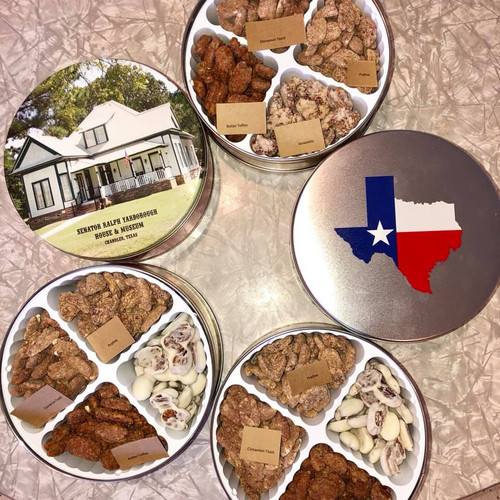The photo shows five circular canisters arranged roughly in a circle on a brown and white marble countertop. Three of the canisters have their lids removed, revealing snacks divided into four compartments per canister; the contents appear to be different varieties of cookies, candied nuts, yogurt-dipped nuts, hard candies, or chocolate pretzels. The two canisters with their lids on are notable for their decorative themes. The canister on the left features an image of a white house with some unreadable commemorative text that indicates it is the house and museum of Senator Ralph Tard located in Cramlin, Texas. The canister on the right displays an outline of the state of Texas, overlaid with the Texas flag. The arrangement and designs suggest these might be commemorative or themed food tins.